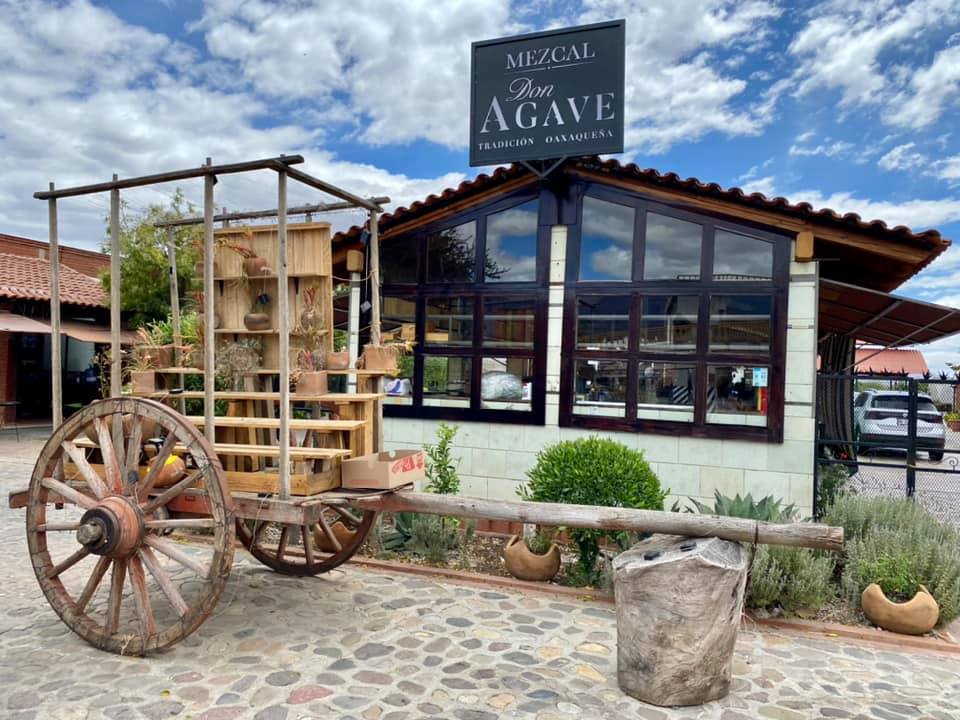This image captures a distinctive, desert-themed setting showcasing a white building with large, uniquely shaped windows framed in dark brown wood. The building features a sign reading "Mezcal Don Agave" and possibly referencing tradition in Spanish beneath, hinting at its connection to the local agave-based beverage culture. The structure, potentially a restaurant or gallery, stands behind a wagon adorned with a variety of plants and pots, indicative of a rustic and old-school aesthetic. The wagon, with its prominent wheels and wooden shelving, adds to the vintage charm, resting one of its spokes on a boulder. Surrounding the building are several drought-resistant plants, complementing the cobblestone-patterned ground. An SUV is parked to the right of the scene, and the whole setting is bathed in the bright, clear light of a desert with a backdrop of blue sky and scattered clouds, enhancing its arid, Mexican vibe.